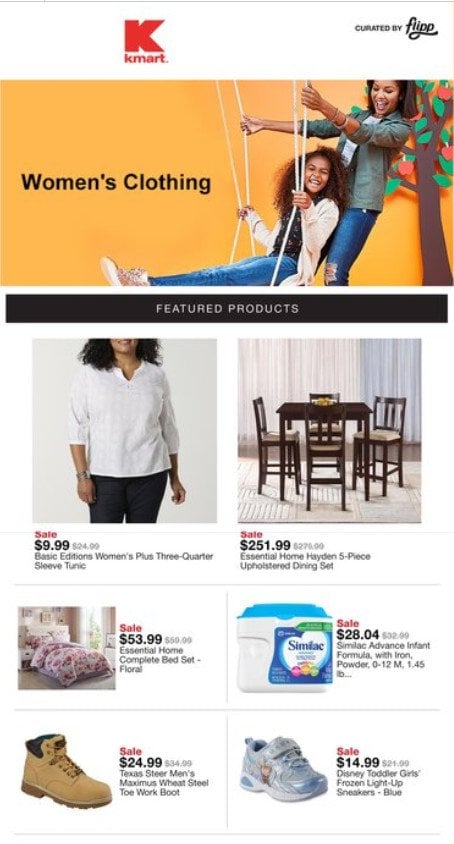The image depicts a Kmart advertisement featuring various products. On the upper left side of the image, there's the recognizable Kmart logo, consisting of a large red "K" with "Kmart" written below it. To the right of the logo, the caption "Curated by Flippa" appears, emphasizing that the selection is specifically chosen. Beneath, a large yellow rectangle highlights women's clothing, featuring an illustration of a mother pushing her daughter on a swing. Behind them, a cutout tree made to look like it's crafted from construction paper adds a charming, whimsical touch. In black text on the yellow background, it reads "Women's Clothing."

A black band below the image contains the words "Featured Products" in white font. Below this header are various product advertisements. 

- On the left: An image of a woman wearing a shirt with a sale tag stating "$9.99, was $24.99." The description reads "Basic Editions Women's Plus Three-Quarter Sleeve Tunic" in gray text.
- To the right: An image of a dining room set featuring four chairs and a table. The sale price is $251.99, down from $276.90, labeled as the "Essential Home Hayden Five-Piece Upholstered Dining Set."
- Below on the left: An advertisement for a "Complete Bed Set" from Essential Home, with a sale price of $30.99, reduced from $59.99, described with a floral design.
- To the right: Promotion for "Similac Advance Infant Formula with Iron," on sale for $28.04, previously priced at $32.99. 

The clean, detailed layout of the advertisement effectively showcases Kmart's diverse product offerings.